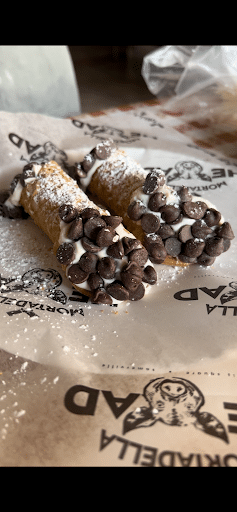In a vividly detailed indoor photograph, two cannolis are elegantly displayed on a sheet of parchment paper. The rectangular image, measuring approximately three inches in height and one inch in width, features thin black headers and footers framing the picture. On the parchment paper, an upside-down image of a pig’s head and some partially legible black text, likely reading "mortadella head," hints at the branding associated with the scene, perhaps suggesting a specialty bakery.

The cannolis themselves are a light, golden brown, stuffed with rich, white cream spilling slightly from both ends, each garnished with a generous number of small chocolate chips. A delicate dusting of powdered sugar enhances their tempting appearance. The photo reveals a bit of the setting: a red and white checkered tablecloth peeks out from underneath the parchment paper, providing a quaint, homey touch, while in the background, a white chair and a glimpse of brown flooring are also visible. The presence of a plastic bag in the upper right corner suggests a busy kitchen environment, and the view of someone possibly wearing a plastic glove further underlines this impression, hinting at the preparation process behind these delectable treats.